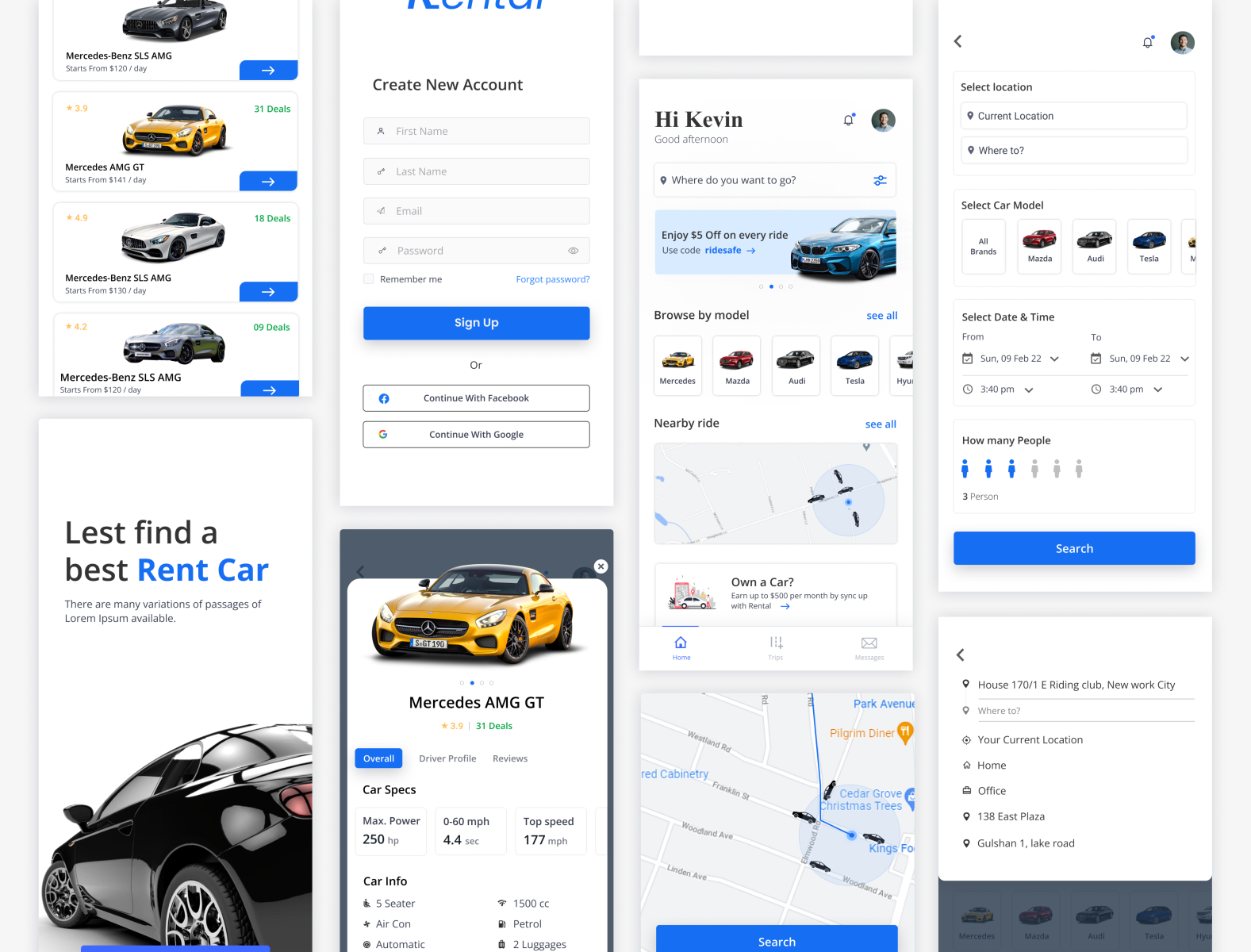**Descriptive Caption:**

The mobile screenshot features several distinct sections of a car rental app. Starting in the top left, there's a section showcasing various Mercedes-Benz cars, including models such as the Mercedes-AMG GT and Mercedes-Benz SLS AMG. Each car is listed with a small image above it, and there is a blue box with a white arrow pointing to the right for more options.

At the top of the screen, there is a cropped blue logo and text reading "Create New Account." Below this, there are fields to fill in personal information and options to sign up with a blue button or continue with Facebook or Google buttons.

Another section of the screenshot greets a user with "Hi Kevin" and offers $5 off every ride alongside a display of car models to select from. There is also a small map indicating nearby rides.

Next, there's a screen with the title "Select Location," where users can input their current location or destination. Options to choose the car model, date, and time are available, along with a selection button for up to six people. A blue "Search" button is prominently displayed.

Adjacent is an image with the text "Let's find the best rent car," accompanied by more details and a picture of a black car.

The final section showcases a selected yellow Mercedes-AMG GT. It provides car specifications and additional information. A map is present beneath the car details, followed by a box containing text that seems to include an address or location information. 

Overall, the screenshot presents a detailed walkthrough of the car rental app, depicting various functionalities and user interface elements.